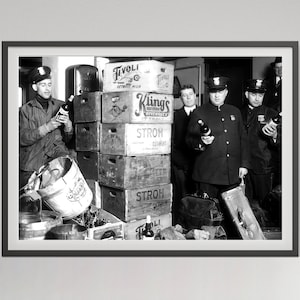This vintage black-and-white photograph, likely from the Prohibition era, captures an intense moment of a police seizure of illegal alcohol. Three police officers, dressed in period-appropriate uniforms complete with police hats, are each holding a bottle of wine and scrutinizing it closely. To the left is one officer, while two others stand to the right. Behind the officers on the right is a fourth man in a suit, whose role is ambiguous but who appears equally engrossed in the examination. The background is dominated by large wooden crates and cases, possibly inscribed with names like "Strau," "Tivoli," and "Klings," suggesting their unknown origins. These crates, likely filled with contraband alcohol, loom from floor to ceiling. In the foreground, scattered containers and bottles further attest to the sizeable stash of illegal liquor seized. The photograph, framed by a white border with an outer black edge, offers a compelling glimpse into a bygone era of law enforcement and illicit trade.